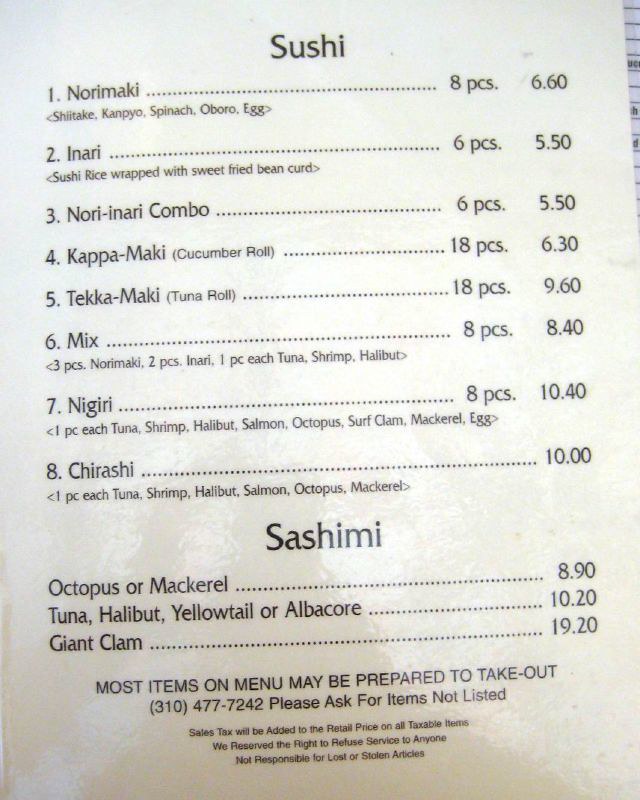This is a detailed caption for the snapshot of a Japanese menu:

The image captures a Japanese menu presented in a minimalist black and white design. The background is white, while the menu text is distinctly black. The menu offers a variety of sushi and sashimi options. There are eight different types of sushi priced between $6.60 and $10. These include:

- **Norimaki:** Shiitake mushroom, kampyo (dried gourd strips), spinach, ogre, and egg rolls.
- **Inari:** Sushi rice wrapped in sweet fried bean curd, provided in six pieces.

For sashimi, the prices range from $8.90 to $19.20, featuring options such as octopus, mackerel, tuna, halibut, and yellowtail.

A note at the bottom of the menu states, "Most items on the menu may be prepared to take out," and includes a phone number for orders, indicating the location is Maryland. Another line reads, "Please ask for items not listed," suggesting additional off-menu selections. Sales tax is noted to be added to the retail price of all taxable items, and the establishment reserves the right to refuse service to anyone. It also mentions they are not responsible for lost or stolen articles. This concise yet comprehensive menu offers a glimpse into the diverse and traditional Japanese cuisine available at this establishment.